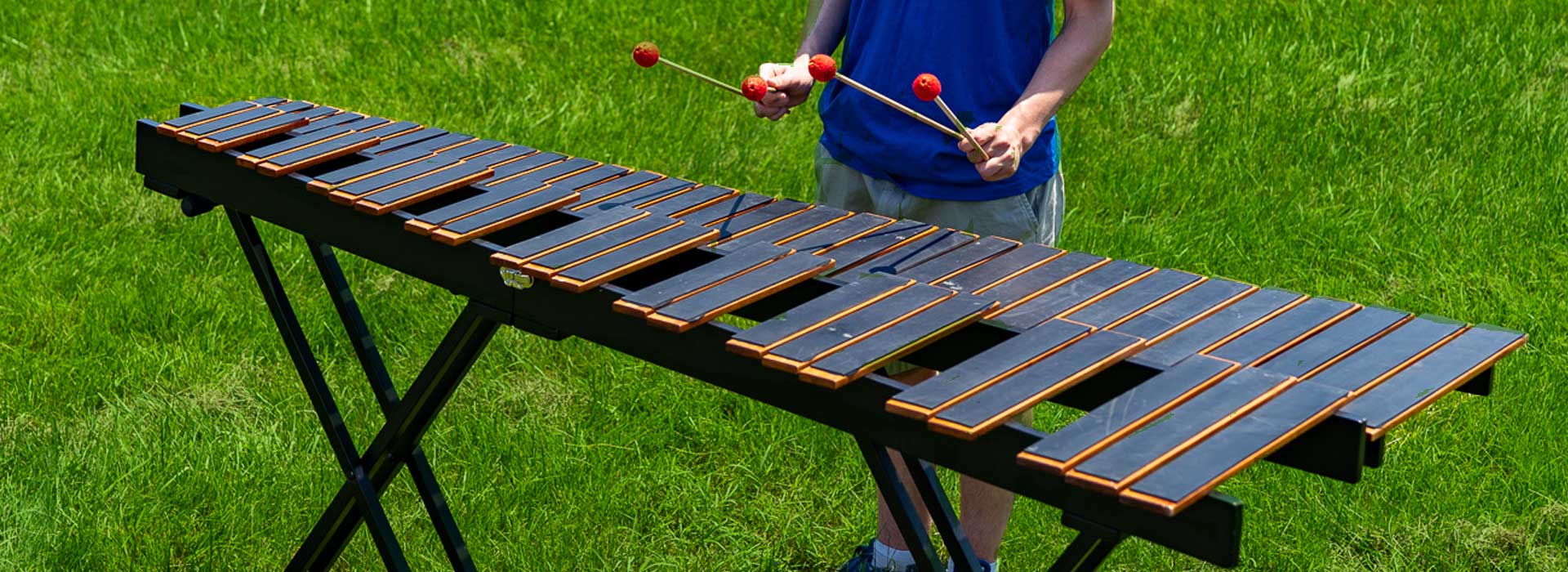An outdoor scene showcases a person playing a large, two-layered xylophone, set up on a lush and slightly overgrown grassy area. The xylophone is approximately six feet long, featuring a distinctive design with a fully populated lower row and an upper row that has noticeable gaps between the bars. The person is dressed in a blue t-shirt, light gray or khaki shorts, and white socks, and is visible from the ankles up to just below the chest. They are holding four mallets, two in each hand, with wooden handles and reddish-orange tips. This suggests a high level of skill. The mallets cast visible shadows on the xylophone's metallic bars, adding a touch of depth to the sunny setting. In the background, the person appears to be alone, surrounded by the vibrant greenery.